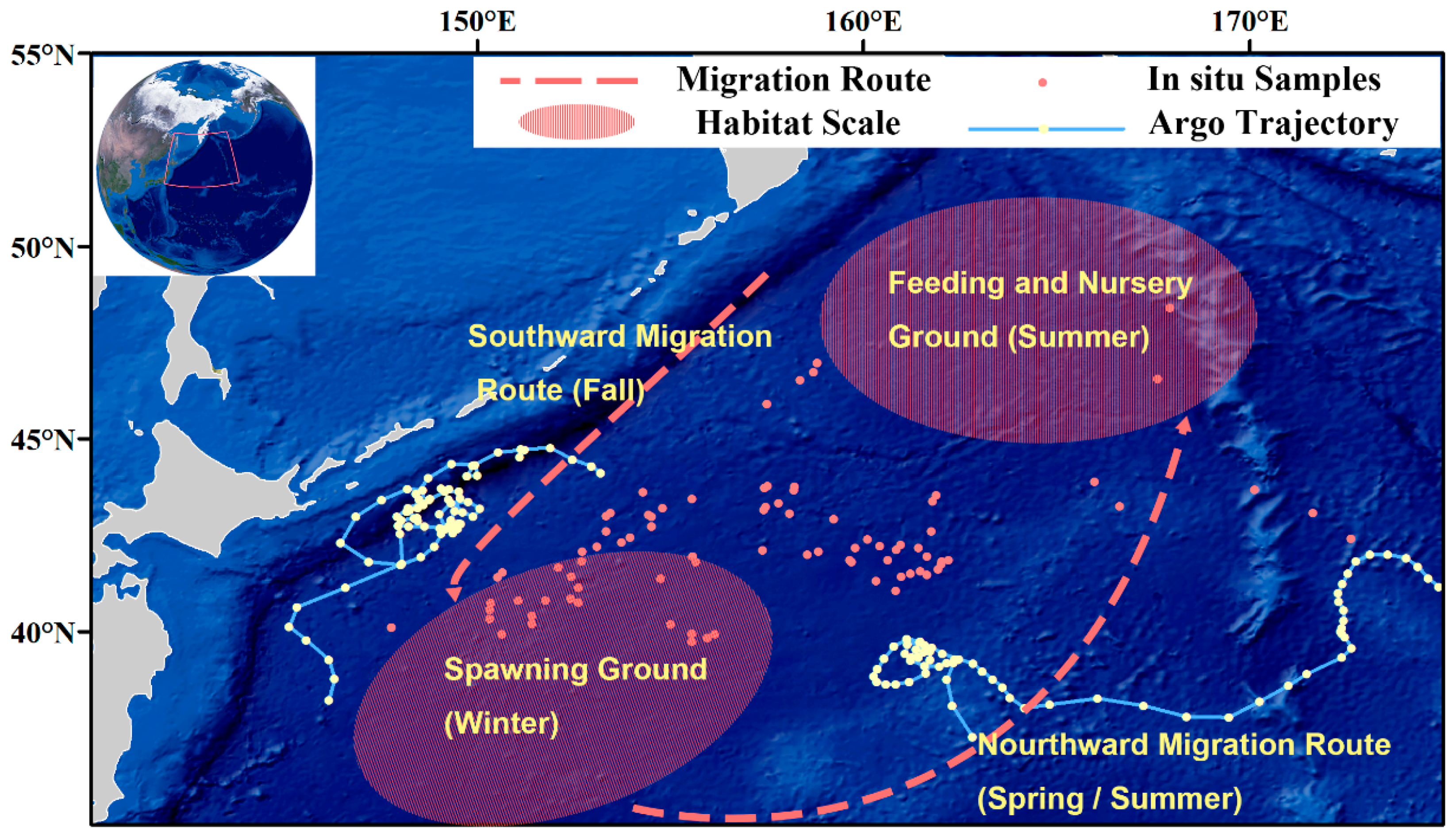The image depicts a detailed map of a specific region, likely in the Pacific Ocean, showing the migration routes, habitats, and seasonal grounds of an unidentified marine species. The majority of the map is dominated by a dark blue color representing the ocean, interspersed with light gray areas indicating islands and land. The map is framed by an x-axis running from 150 degrees east to 170 degrees east and a y-axis spanning from 40 degrees north to 55 degrees north.

In the upper left corner, there is a depiction of the globe highlighting the area of interest. Adjacent to this globe, a white rectangular box labels key elements such as migration routes, habitat scales, in-situ samples, and Argo trajectory.

Two prominent purple ovals mark critical areas: the lower left corner features the "Spawning Ground" for winter, and the upper right indicates the "Feeding and Nursery Ground" for summer. These areas are connected by checkered lines tracking the animal's movement. Yellow-lettered labels denote the "Northward Migration Route" for spring and summer, moving towards the feeding and nursery ground, while the "Southward Migration Route" for fall returns to the spawning ground.

Additional visual details include red dots scattered across the blue background, likely representing in-situ samples or recorded sightings of the species. There are also yellow dots and blue line tracks showing the detailed movements across the sea area, emphasizing the continuous monitoring and tracking of the species' migration patterns.